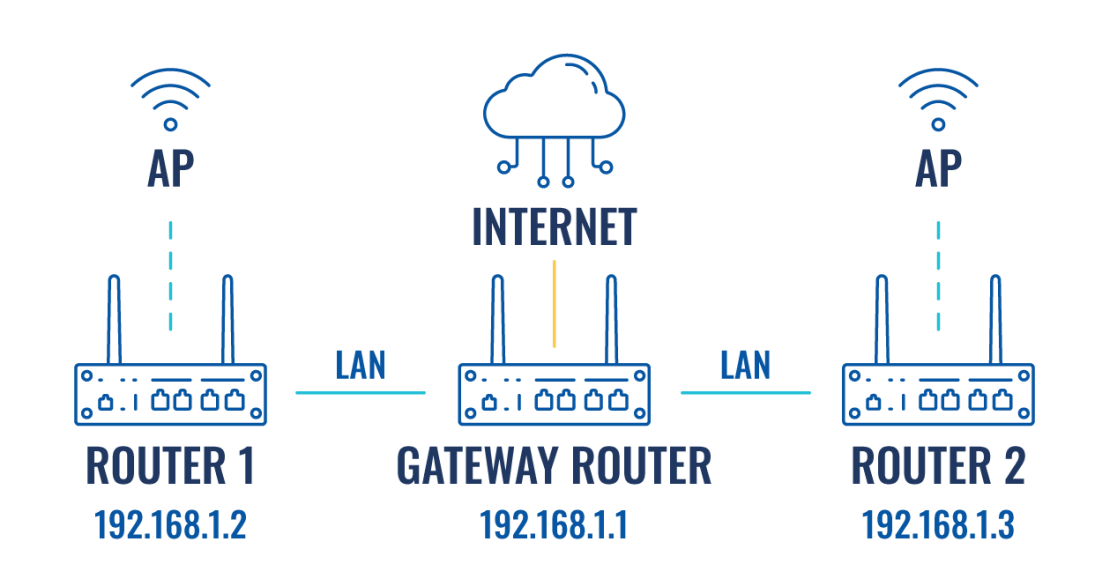The image is a computer-generated diagram illustrating how the internet connects through a series of routers. At the center is the gateway router labeled with the IP address 192.168.1.1, symbolizing its role in connecting to the wider internet, which is depicted as a cloud with lines and dots representing data packets. 

To the left, the diagram shows "Router 1" labeled with the IP address 192.168.1.2, indicated by a Wi-Fi symbol and the label "AP" (Access Point). This router connects to the gateway via a local area network (LAN) line. To the right, "Router 2" is displayed similarly, with an AP label and IP address 192.168.1.3, also connecting to the gateway through a LAN line. The entire depiction is rendered in blue, providing a clear visual representation of how routers interconnect and link to the internet.